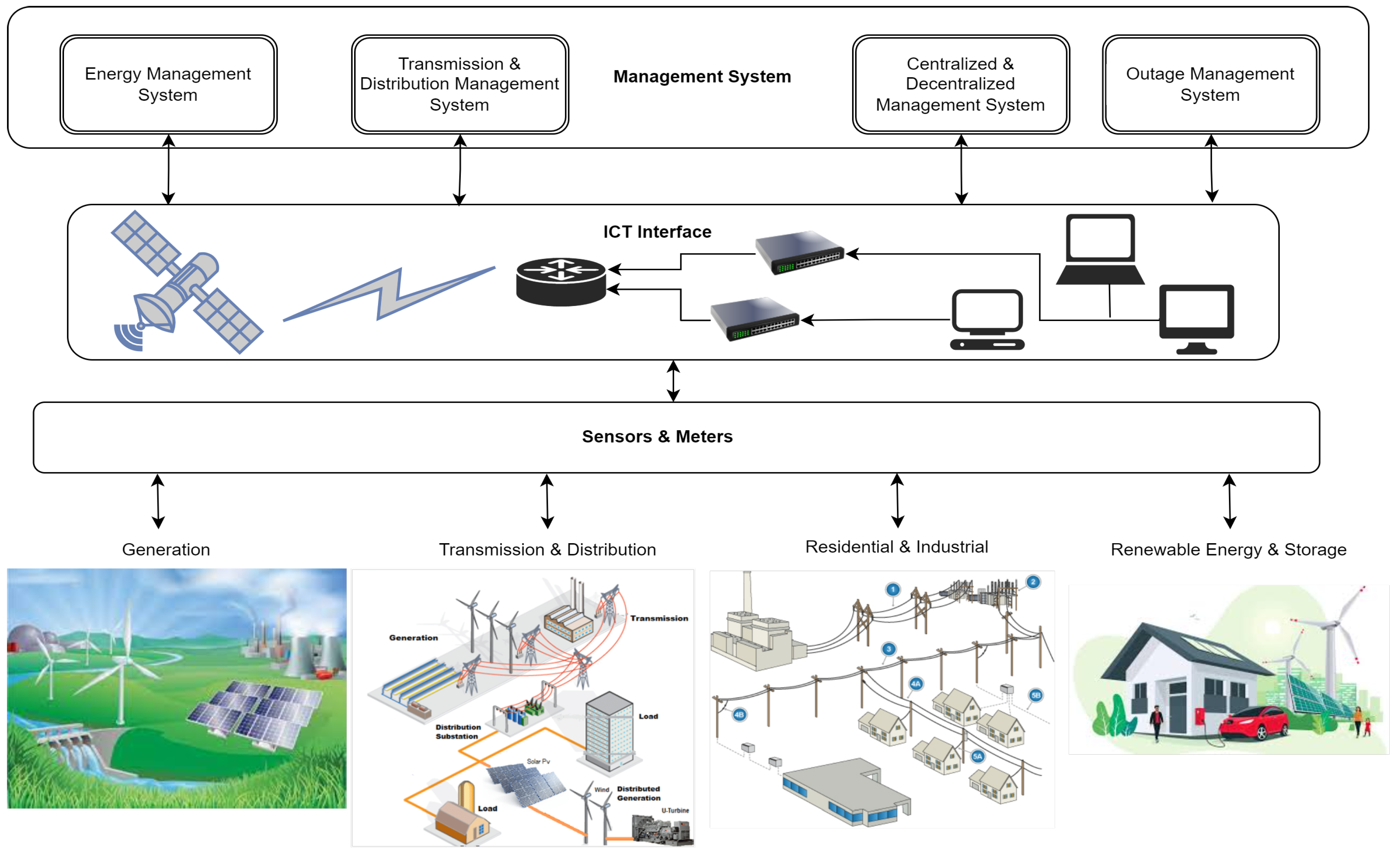The diagram presents a detailed visualization of an energy management system segmented into three principal sections: Management System, ICT Interface, and Sensors and Meters. These sections are interconnected by arrows illustrating the workflow among various components. The management system encompasses sub-systems such as Emergency Management System, Transmission and Distribution Management System, Centralized and Decentralized Management System, and Outage Management System, establishing a comprehensive framework for energy management. Central icons include a satellite, a lightning bolt, and ICT interface devices. At the bottom, four pictures depict different stages of energy flow: generation represented by a power plant, transmission through farmlands and solar panels, and distribution to residential and industrial areas. The diagram underscores how information flows seamlessly from satellites to various sectors to maintain communication and manage electrical systems efficiently, particularly during outages.